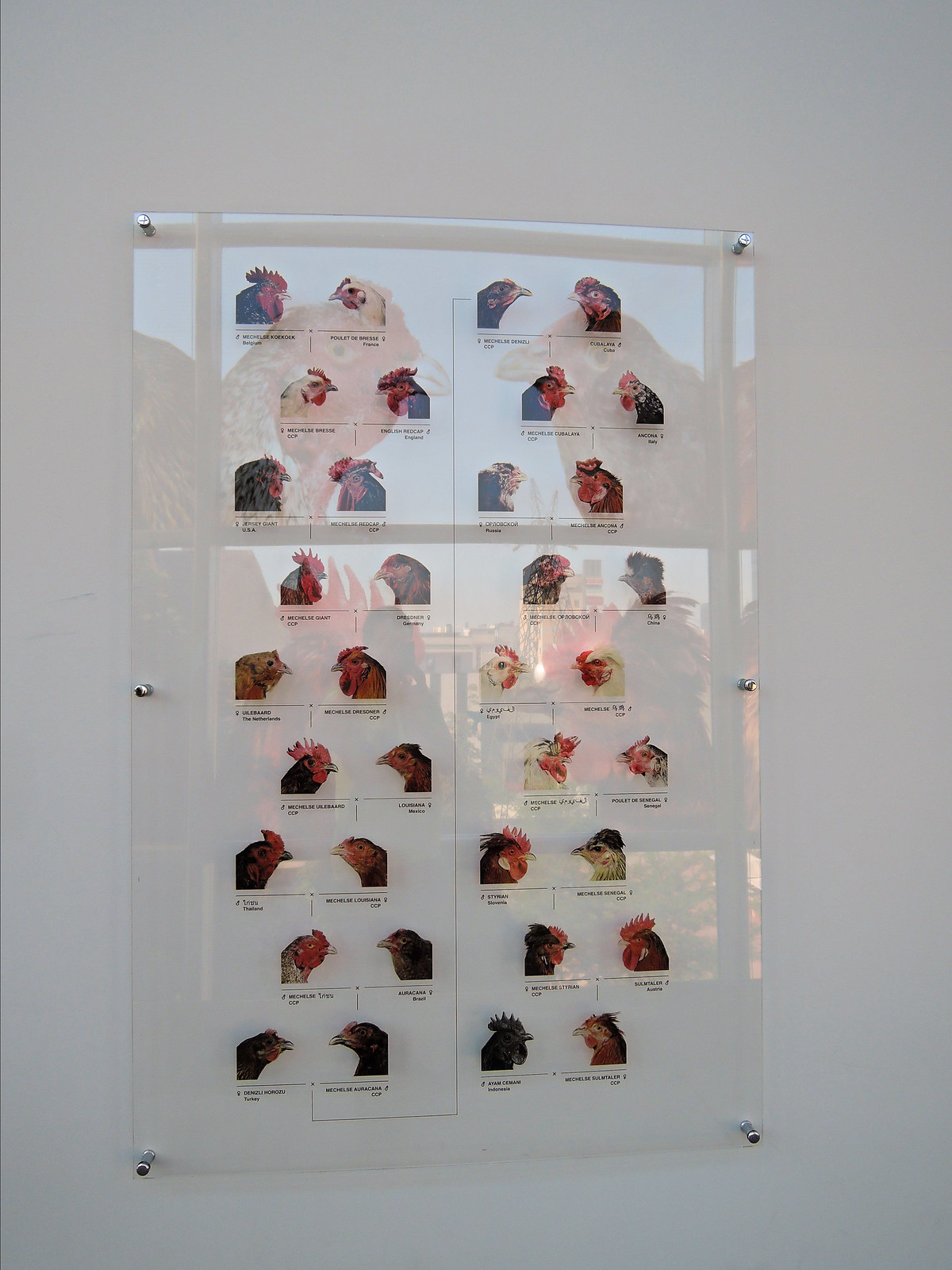The photograph captures an instructional display mounted on an off-white, light gray gallery wall. The display is encased in a large sheet of clear, acrylic plastic, affixed securely with six chrome or steel screws positioned at the top corners, bottom corners, and midway along the sides. The display features a comprehensive collection of headshots showcasing various chicken breeds, roosters, and guinea hens in vibrant colors. These thumbnail-sized headshots are meticulously arranged in rows, each paired with its respective opposite sex, with males generally facing left and females facing right. Each bird is identified by a label beneath its image. Behind these smaller, detailed headshots, the background subtly features faint, translucent, larger images of birds, including roosters with vivid red combs, and hens of bluish or blackish hues. The display serves as an interpretative or educational aid, possibly tailored for a poultry dealer or enthusiast, emphasizing the anatomical and coloration differences among the bird types displayed.